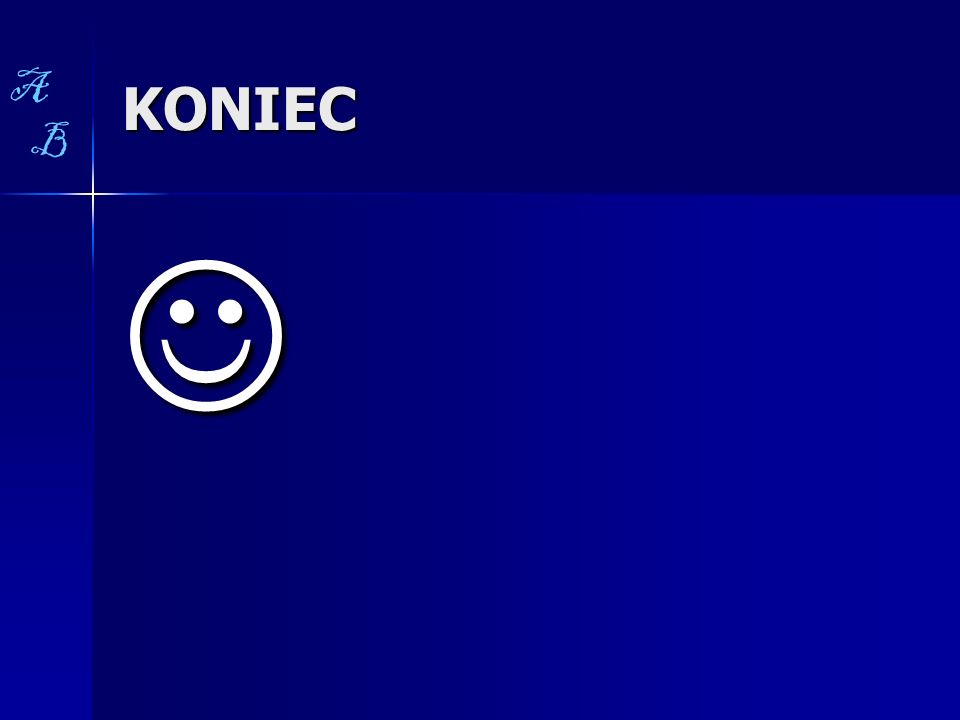The image appears to be a PowerPoint slide with a predominantly blue background that transitions from a darker blue at the top to a lighter blue towards the bottom right and bottom left. The top portion of the slide features a horizontal rectangle section filled with this darker blue. In the upper left-hand corner, there are decorative cursive letters "A" and "B" in light blue. To the right of these letters, the word "K-O-N-I-E-C" is prominently displayed in bold, white, all-caps letters, left-aligned within the darker blue title area. Below this text, in the main lighter blue section of the slide, is a white outlined smiley face, also left-aligned, featuring two filled-in dots for eyes and a curved line for the mouth. The slide has a minimalist and clean design, with a thin border separating the darker top section from the lighter bottom section.